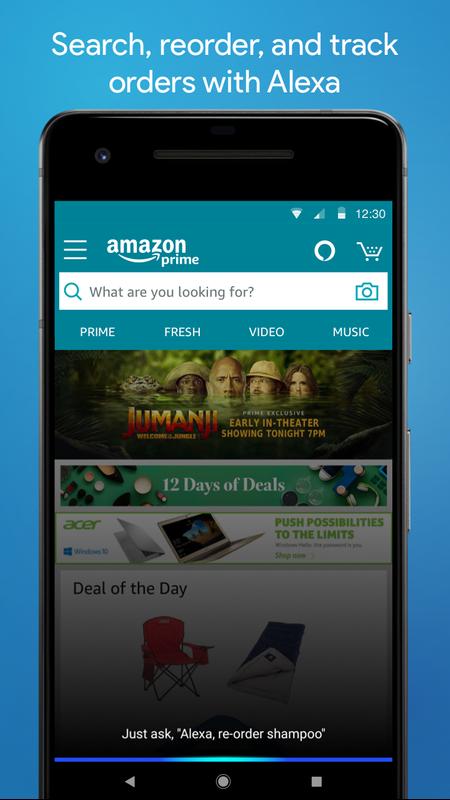**Caption:**

The image showcases a smartphone screen open to the Amazon Prime app. At the top, in white font, is the text "Search, reorder, and track orders with Alexa." The Amazon Prime logo is centered at the top of the screen, flanked by a menu icon with three horizontal lines on the left and a shopping cart icon on the right. Directly below this, a white search bar asks, "What are you looking for?" and includes a small camera icon on its right side, allowing users to search via photo. 

The app's main menu options—Prime, Fresh, Video, and Music—are arranged horizontally below the search bar. The majority of the screen is dominated by visual content, including an advertisement for the film "Jumanji," highlighted with the text "Early in Theaters." Beneath the Jumanji ad, a banner reads "12 Days of Deals."

Following this, there is a featured advertisement for Acer, showcasing a laptop with the slogan "Push possibilities to the limit." Next, the "Deal of the Day" section displays beach chairs at a discounted price.

At the screen's bottom, in white font, is the prompt "Just ask Alexa to reorder shampoo," accompanied by a visual representation of voice waveforms. Three navigational icons are aligned at the bottom: a triangle pointing left (to go back), a circle (likely representing the home button), and a square (perhaps for multi-tasking or recent apps).